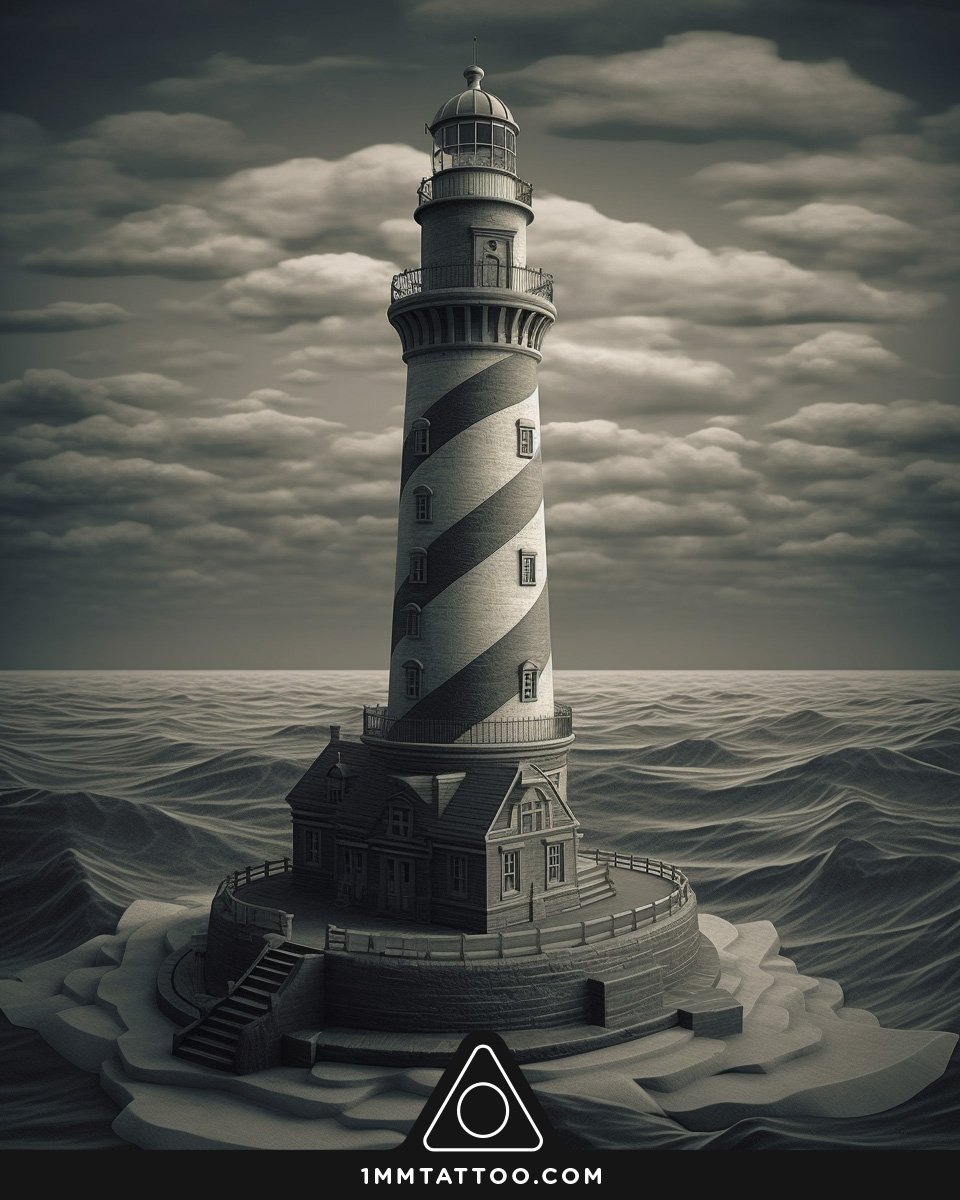This grayscale image, possibly designed for a tattoo, features a prominently detailed lighthouse situated on a small island surrounded by churning ocean waves. The scene is dominated by a cloud-filled sky halfway up the background, adding to the dramatic atmosphere. A stone path leads to the lighthouse, emphasizing its central position. At the bottom of the image, a black stripe spans the width, showcasing a triangle with a white circle inside, beneath which the text "1MMTATTOO.COM" is clearly displayed. The artwork is depicted in a realistic yet somewhat cartoonish style, reminiscent of a finely detailed painting, with all elements rendered in various shades of gray, white, and black, entirely devoid of color.